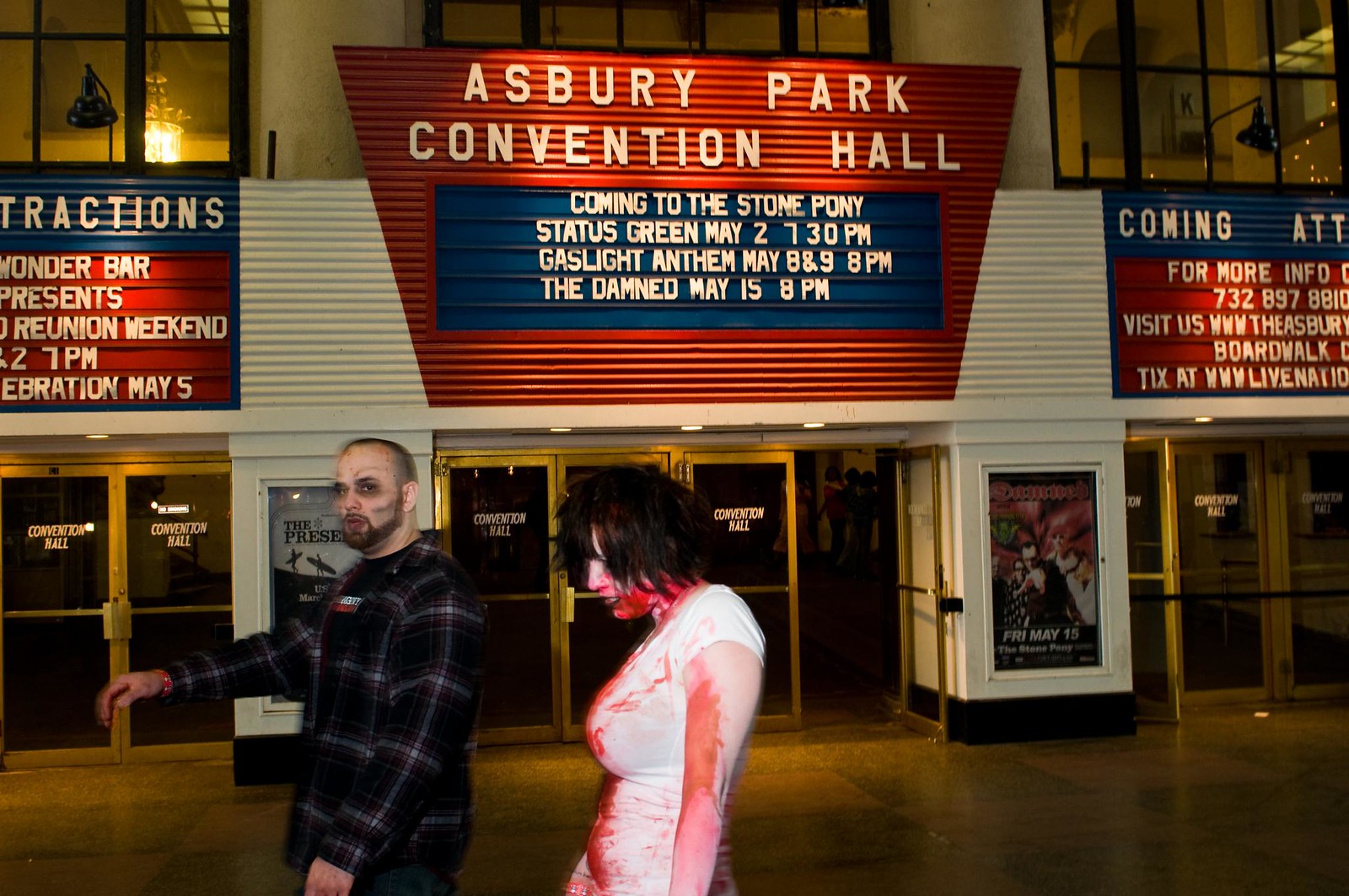In this detailed image, two people are walking in front of the Asbury Park Convention Hall. The building is identifiable by its prominent signage: a large red sign with white letters reading "Asbury Park Convention Hall," and a central blue banner advertising upcoming events. The blue sign announces, "Coming to the Stone Pony: Status Green, May 2nd, 7:30 p.m.; The Gaslight Anthem, May 8th and 9th, 8 p.m.; The Damned, May 15th, 8 p.m." Below the signs are numerous glass doors framed in gold. 

The two individuals appear to be in some form of costume or theatrical attire, perhaps for a themed event. The man, to the left, has a short beard and mustache, is almost bald with thin hair, and wears a black, long-sleeved, plaid shirt with red and white stripes. His face has black lines and appears to be smeared with blood, giving him a zombie-like appearance. The woman next to him, with shoulder-length shaggy black hair, is dressed in a short-sleeved white t-shirt also covered in blood, and her face is similarly stained. They walk in sync, seemingly participating in a Halloween or horror-themed event outside this historical convention hall.